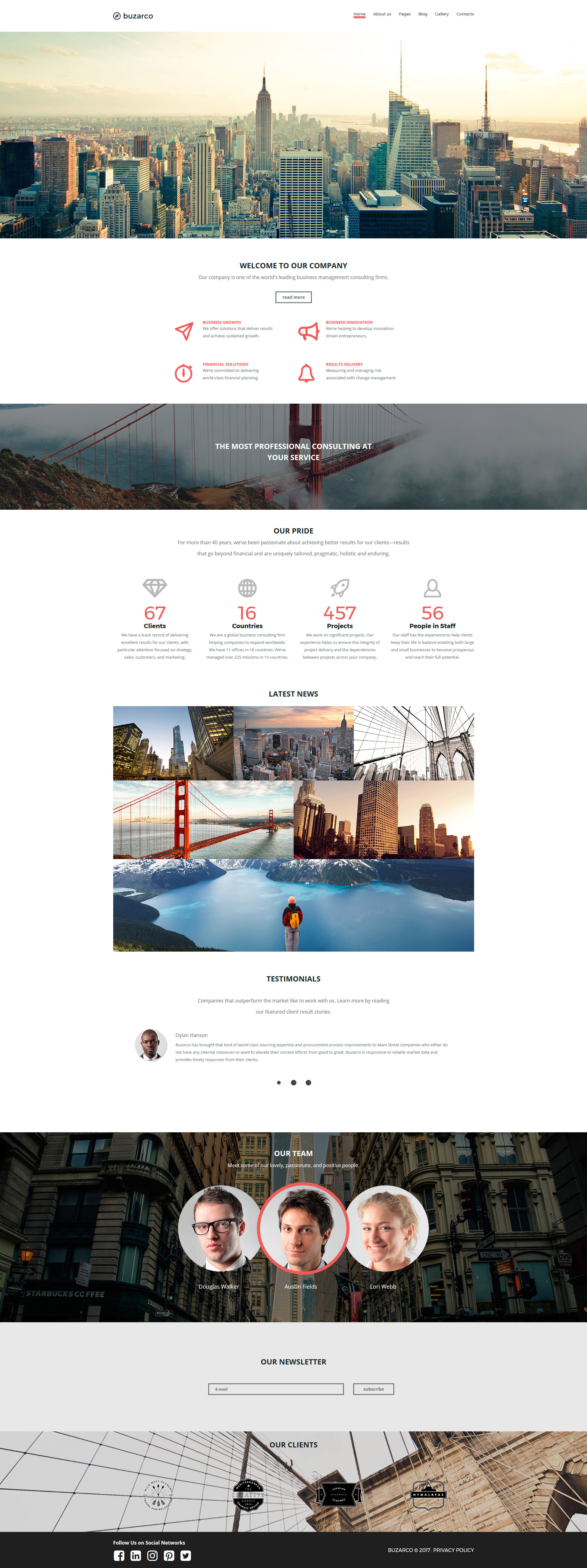In this detailed image, we are looking at a full-length screenshot of the Buzarco website, clearly spelled B-U-Z-A-R-C-O. At the top of the page, the navigation menu is visible, providing links to various sections such as Home, About Us, Pages, Blog, Gallery, and Contacts.

Prominent at the top is a large, striking landscape image of New York City, setting an urban and professional tone. Below this header, a welcoming section introduces Buzarco as a leading business management and consulting firm. The welcoming message reads: "Welcome to our company. Our company is one of the world's leading business management and consulting firms."

Following this introduction, there are several informative links detailing the firm’s core services:
- **Business Growth:** "We offer solutions that deliver results and achieve sustained growth."
- **Financial Solutions:** "We're committed to delivering world-class financial planning."
- **Business Innovation:** "We’re helping to develop innovation-driven entrepreneurs."
- **Results Delivery:** "Measuring and managing risk associated with change management."

As one scrolls down the page, various images of American cities enhance the visual experience. Notably, there is an image of the iconic Golden Gate Bridge in San Francisco, along with multiple images showcasing different views of New York City.

Towards the bottom of the webpage, there is a section featuring the Buzarco team members, presenting a few key staff members who drive the company's success.